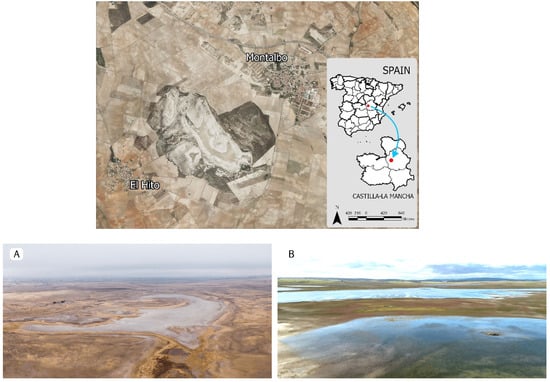This composite image features three distinct photos set against a predominantly white background. The largest photo, positioned at the top, is an aerial shot, possibly taken by satellite, showcasing a predominantly brown and sandy landscape labeled "Montalvo," with "Spain" indicated on a sidebar map. The terrain appears largely undeveloped, although there might be a solitary building near the sidebar, suggesting it could be agricultural land or sparsely inhabited. Below this aerial shot are two panoramic images labeled "A" and "B," seemingly captured from an airplane. These images depict substantial bodies of water, with notable features suggesting they could be lakes that are in the process of drying up. Sandy and flat areas are visible in both shots, reinforcing the impression of a desiccated landscape.